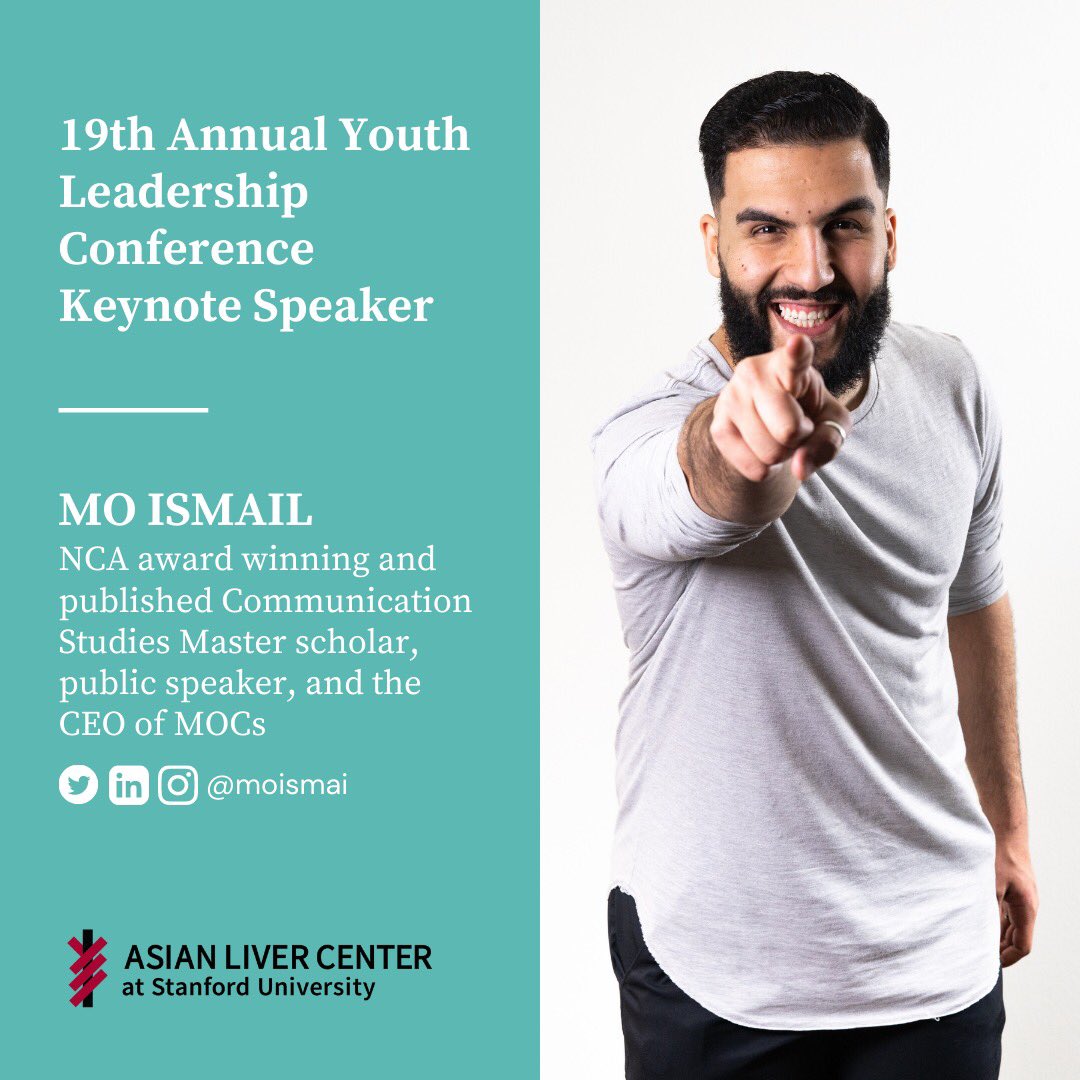The image is a detailed advertisement for the 19th Annual Youth Leadership Conference. It is divided into two parts, with the left half featuring a background in Tiffany blue. This portion includes white text that reads: "19th Annual Youth Leadership Conference Keynote Speaker, Mo Ismail, NCA Award-Winning and Published Communication Studies Master Scholar, Public Speaker, and CEO of MOCs." Additionally, it displays social media symbols for Twitter, Instagram, and LinkedIn, and mentions "Asian Liver Center at Stanford University" at the bottom.

The right half of the image has a white background and showcases a man standing and pointing directly at the camera with his index finger, reminiscent of the Uncle Sam "I Want You" pose. The man has short black hair, a short black beard with a mustache, and is wearing a long-sleeved gray or white shirt paired with black pants. His appearance suggests Middle Eastern or South Asian ethnicity, and he is portrayed smiling warmly.